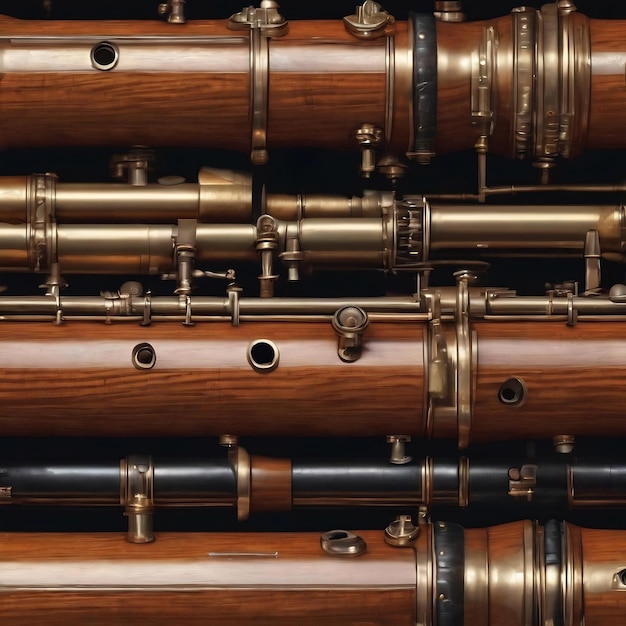In this detailed photorealistic image, several cylindrical objects, resembling pipes with a steampunk aesthetic, are arranged horizontally against a dark black backdrop. The image prominently features three main brown wooden cylinders, adorned with bronze and black accents. These wooden cylinders have multiple holes lined with bronze, enhancing their intricate, mechanical appearance. 

The topmost cylinder is made of brown wood, wrapped with bronzy accents that attach it to a smaller bronze cylinder beneath. This middle bronze cylinder, adorned with various attachments and appendages, connects to another brown wooden cylinder, which features more holes and a prominent bronze rod running lengthwise along its top.

Further down, this wooden cylinder connects to a slender black metal cylinder, accented with wood and brass. At the very bottom, another brown wooden cylinder is visible, characterized by black and brass accents as well as additional holes.

The overall composition, with its shiny, well-maintained surfaces and complex interconnections, evokes a steampunk vibe, making it unclear whether these objects are part of musical instruments or some kind of machinery. The image's close-up view emphasizes the detailed craftsmanship and the intriguing fusion of materials like wood, bronze, and iron, creating an enigmatic yet visually captivating scene.